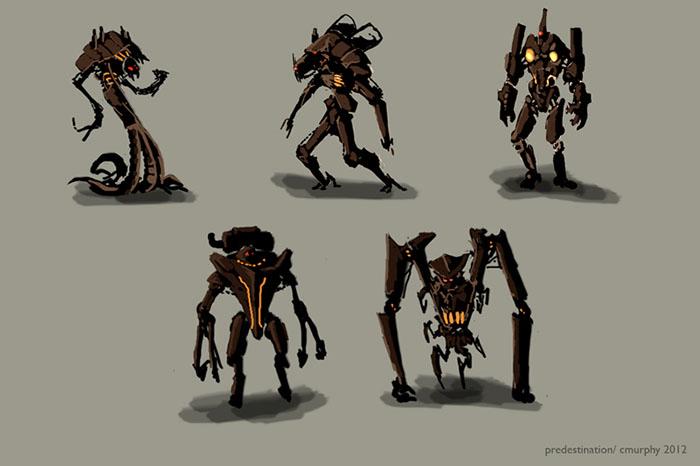The digitally generated graphic image features a collection of five eerie, alien robot-like characters set against a completely gray background. The only text present, located in the bottom right corner in small, dark gray print, reads "Predestination/Seamurphy 2012." Positioned in a 3-by-2 arrangement, three characters are aligned at the top and two at the bottom.

At the top left, there is a brown creature with red eyes and a highly curved, somewhat octopus-like body structure. The middle character is also dark brown and has an elongated head reminiscent of 1980's battle bot animation. The top right figure stands out with a pointier head and a few yellow marks on its chest.

On the bottom row, the character on the right is spider-like, featuring long wings or arms that reach the ground, red eyes, and extensive yellow areas around the belt. The figure to the left complements the lineup, resembling a mechanical robot with a split head, significant misshapen limbs, and a body that hints at both organic and machine elements.

All characters share segmented, abstract structures, presenting a haunting fusion of humanoid and animalistic designs, highlighted primarily in shades of brown and black, with occasional gold accents, thus enhancing their sinister appearance.